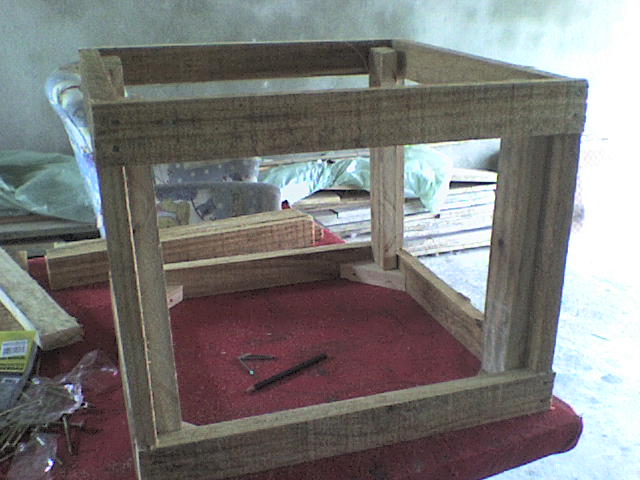The photo appears to have been taken inside a garage or workshop, showing a cluttered workspace filled with woodworking materials and tools. The focal point is a wooden structure, resembling a small end table or toy box frame, flipped over on a table. The frame has no sides, just an exposed wooden box reinforced at the joints. The table beneath it is draped with a red covering, possibly a cloth or tarp. Inside the frame, there are a couple of nails and a carpentry pencil.

To the left of this wooden structure, there is a ripped-open bag with nails scattered about. The background reveals a haphazard collection of wooden planks and plywood, indicating ongoing construction or woodworking projects. A small armchair with blue and white designs, likely a child's chair or a workshop chill-out chair, is visible amidst the clutter. The workshop has concrete floors and walls, adding to its utilitarian atmosphere. The overall scene suggests a busy, active space dedicated to building or remodeling, filled with the necessary materials and tools for various carpentry tasks.